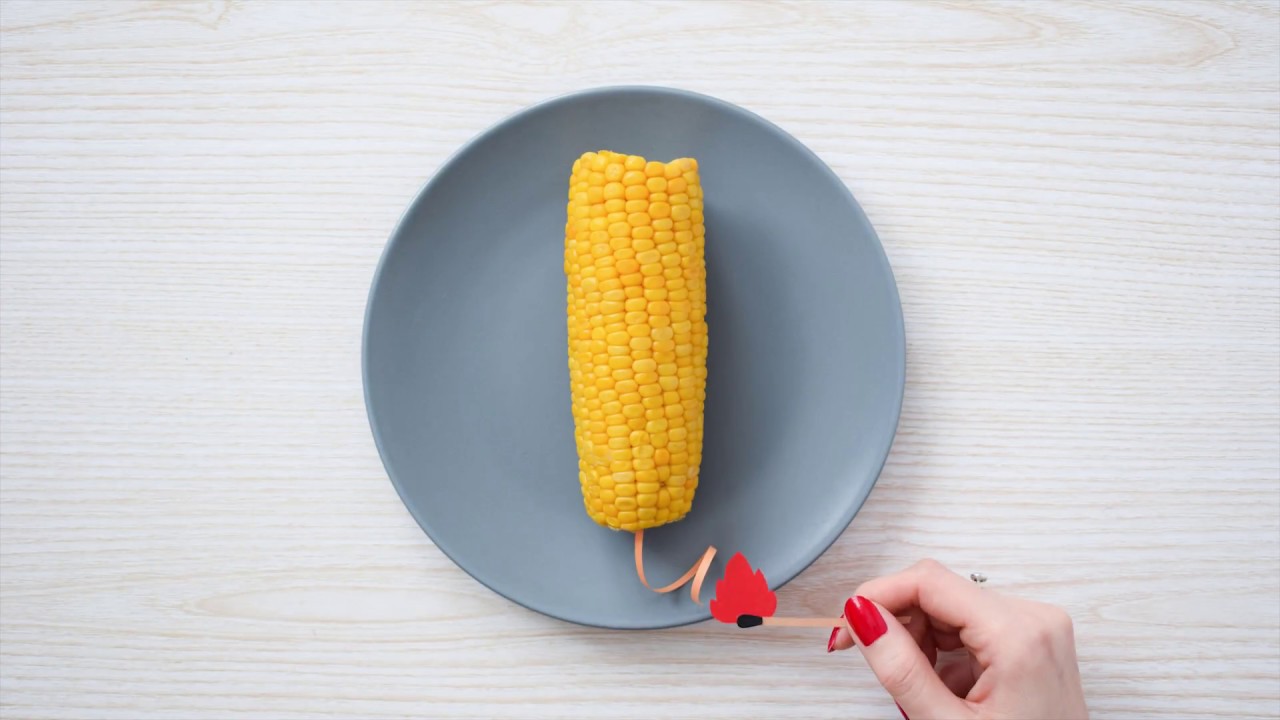In the center of the image, there's a light bluish-gray, round plate placed on a light wooden surface with horizontal wood grains. Vertically aligned on the plate is a yellow ear of corn. Attached to the bottom of the corn is a curly, light pink ribbon, resembling the fuse of a dynamite stick. A female hand with red-painted nails and a visible ring is holding a match towards the ribbon, coming in from the bottom right of the image. The match has a black tip and a red flame, but it's a paper illustration rather than a real match. The entire scene creates the illusion that the hand is about to ignite the ribbon, mimicking the action of lighting fireworks.